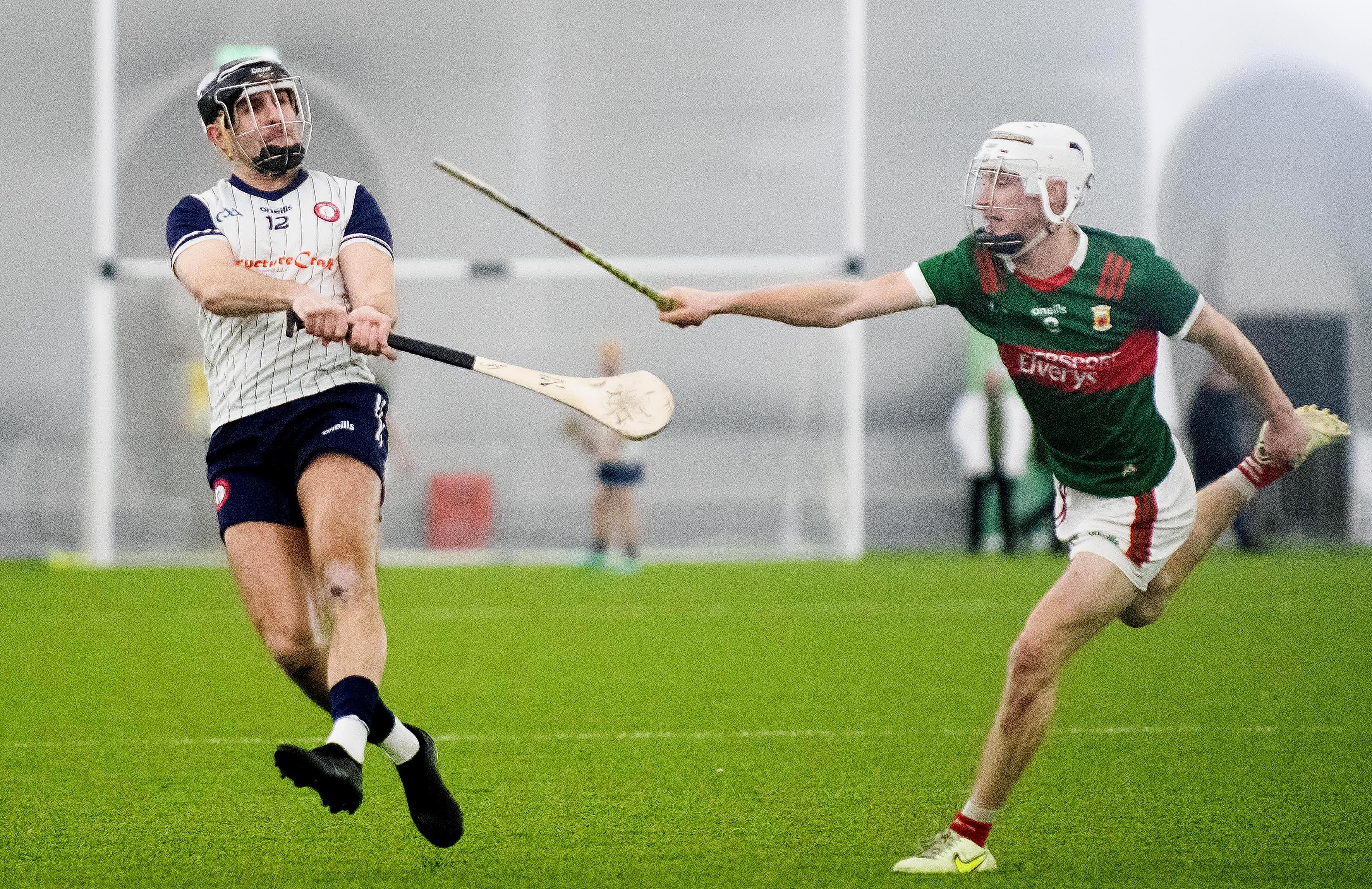This vibrant photograph captures a dynamic moment between two lacrosse players on a field, characterized by bright green grass under an overcast sky. The player on the left wears a predominantly white jersey adorned with blue stripes and blue sleeves, paired with black shorts, black cleats, and white and black socks. He grips a lacrosse stick, distinguished by its flat end, positioned as if ready to engage with an unseen ball. The player on the right, clad in a green jersey with red print across the chest and red stripes on the shoulders, complements his top with white shorts featuring green and red stripes down the side, white cleats, and red and white striped socks. He mirrors a similar engaged stance, extending his own lacrosse stick, seemingly set to intercept or challenge his opponent. Both players wear protective helmets with face masks, further emphasizing their intense involvement in the game. In the misty background, a goalkeeper stands vigilant in front of a net, under the gray, cloud-filled sky, adding depth and context to this vivid sporting scene.